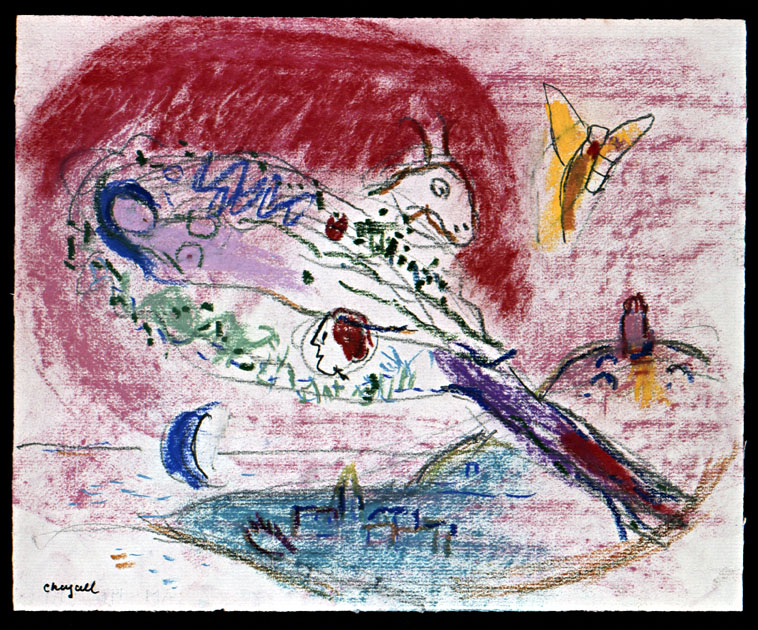The image depicts a painting with a black border framing an abstract, childlike composition. It features rudimentary and whimsical elements, which suggest it could be either a chalk drawing, pastel work, or a light-painted canvas. Central to the artwork is an oblong shape, outlined in green and blue, possibly representing a woman or mermaid, with distinctively green-lined breasts and blue hair. Adjacent to her is a rudimentary animal figure—potentially a ram, dog, or horse—hovering above what appears to be a body of water. The background is energetically marked with swathes of red, as though the brush was dancing across the canvas. A mass or island lies below the central figures, topped by a pink sky that adds to the painting's dreamlike quality. To the right, a fairy-like or butterfly figure flits across the scene, colored in golden hues, contributing to the fantastical atmosphere. In the upper regions, more whimsical creatures like a primitive bird or butterfly can be seen, while near the bottom, a village or castle on a hill sits near what seems to be a lake or sea. The entire scene conveys a spontaneous and vibrant narrative, imbuing a sense of innocence and imagination that echoes styles reminiscent of Marc Chagall's work, or perhaps another artist with a similar signature.